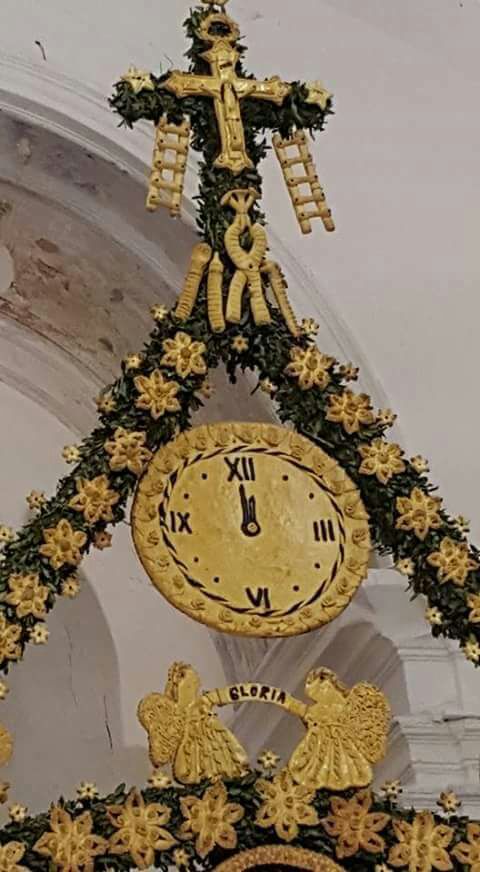A beautiful and ornate religious decoration is on display, resembling something one might find in a church setting. It features a green vine wreath adorned with a variety of intricate elements. At the top of the wreath, a gleaming gold cross is prominently positioned, with a star on each end of the crossbar. Surrounding the cross, lush greenery cascades down, with two ladders hanging from each side, symbolizing ascension. Below the cross, additional golden ornaments dangle, adding to the decoration's opulence. The greenery extends outward from the sides, with vibrant flowers interwoven into the foliage, creating a striking visual effect.

In the central part of the wreath, nestled between the greenery, is a clock with an antique look, displaying Roman numerals. The clock face highlights only the numbers 12, 3, 6, and 9, adding a classic touch to the piece. Beneath the clock, two elegant golden angels stand facing each other, holding an arched banner inscribed with the word "Gloria." The angels and the banner form a harmonious and spiritual accent to this exquisite display, evoking a sense of divine glory and reverence.